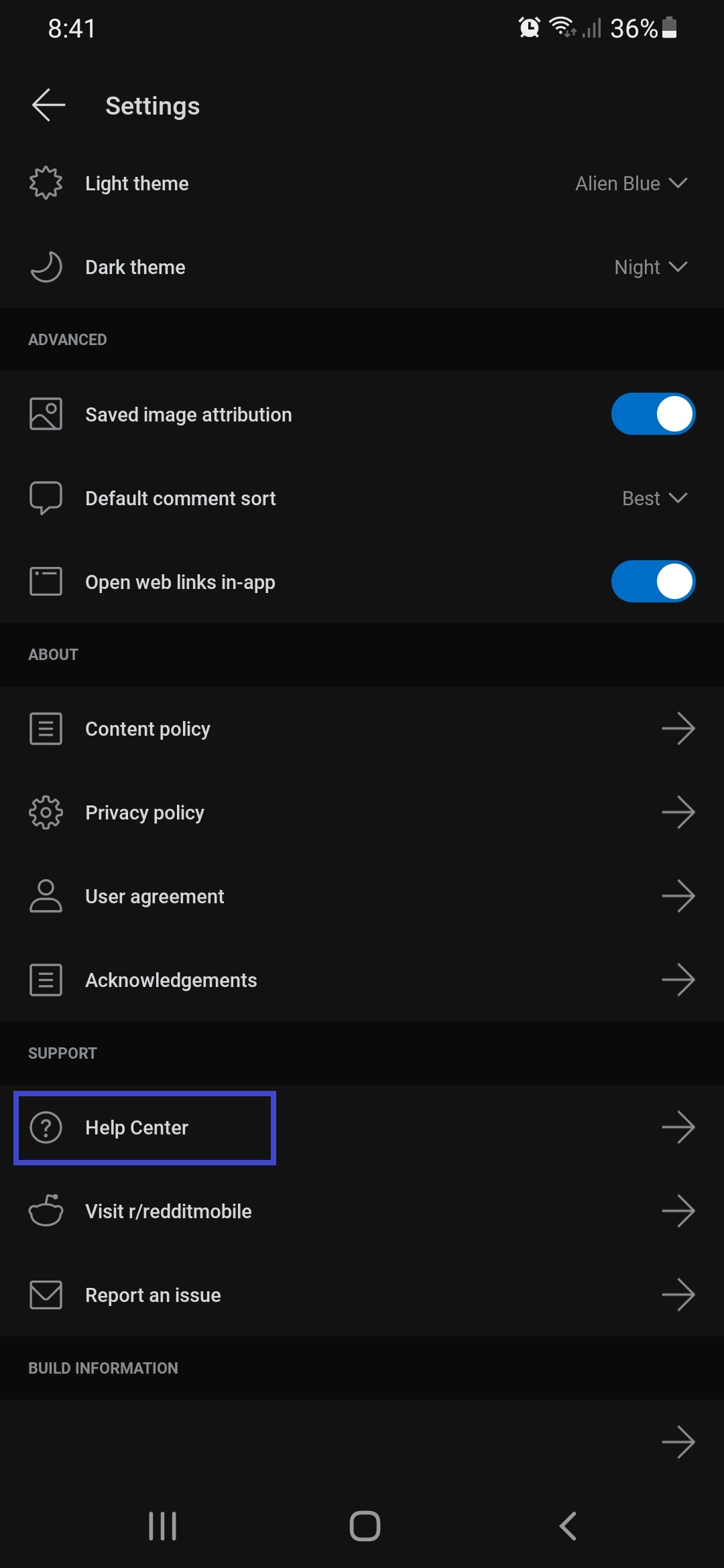A detailed screenshot of a cell phone screen displaying a settings menu. The screen has a black background, with the time "8:41" visible in the upper left corner and a battery level of 36% indicated nearby. Despite having no service bars, an online indicator is present. An analog clock appears in the upper right corner. 

The menu consists of several items:
- "Light Theme" with a gear icon.
- "Alien Blue," indicating a setting choice.
- "Dark Theme" marked as "Night," reflecting the current screen's appearance.
- "Advanced" settings.
- "Saved Image Attribution," turned on.
- "Default Comment Sort" set to "Best."
- "Open Web Links in App," activated with a switch turned to the right.
- "Content Policy" with a right arrow.
- "Privacy Policy" marked by a gear icon and a right arrow.
- "User Agreement" with a right arrow.
- "Acknowledgements" also featuring a right arrow for more options.

Support options include:
- "Help Center," bordered in blue with a question mark icon and a right arrow.
- "Visit Our Reddit Mobile" with a right arrow for further information.
- "Report an Issue," marked by an envelope icon and a right arrow.

Finally, "Build Information" with a right arrow.

At the bottom of the screen, three navigation icons are visible: three vertical lines on the left, a circle in the center, and a left-facing arrow in the lower right corner.